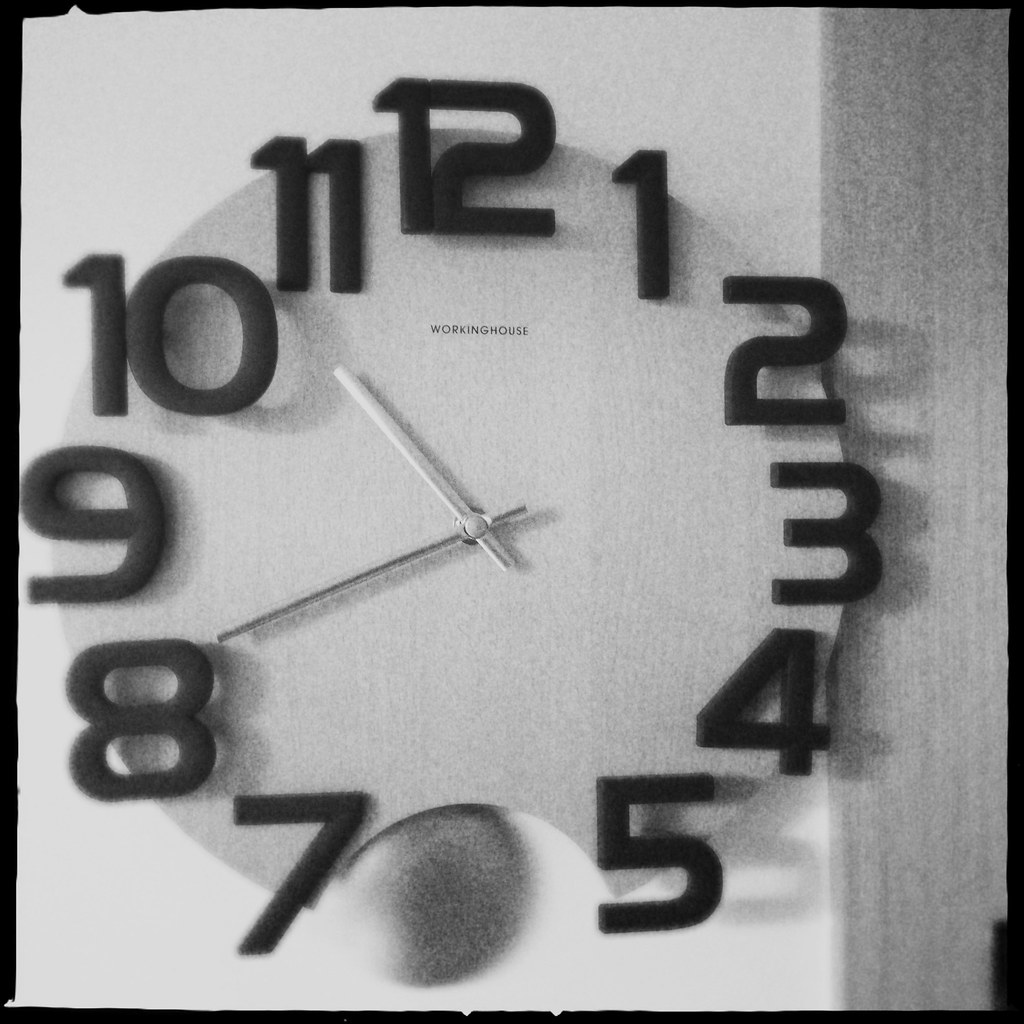A close-up, black and white photograph of a clock prominently framed within black lines. The clock face is a light grey circular shape, from which a semicircular wedge has been cut out at the bottom. Through this removed section, a fuzzy pendulum, rendered in darker grey, dangles down. The clock features bold, black numerals from 1 to 12. However, the number 6 is absent due to the cutting of the wedge. The clock’s hands are grey and lack a second hand, only displaying the hour and minute. Below the number 12, the words "WORKING HOUSE" are printed in small black text.